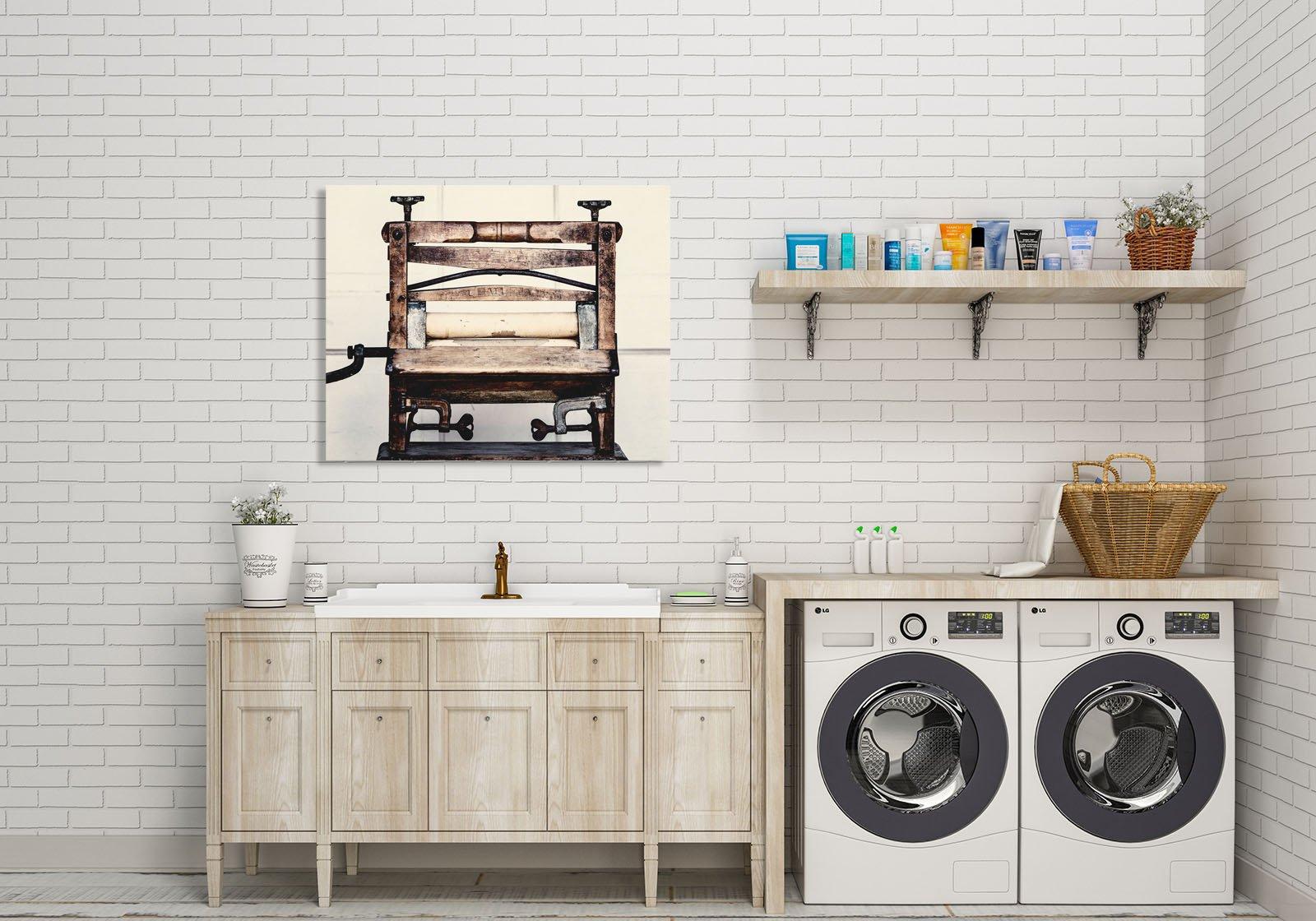This image features a meticulously arranged laundry room with a clean and modern aesthetic. The back wall is adorned with a white brick-patterned wallpaper that looks almost too perfect to be actual brick, lending a uniform and clean look to the space. Dominating the lower portion of the room are two front-loading white washing machines nestled under a light wood veneer countertop. The countertop above the machines serves as a utility space, holding a laundry basket and a variety of other items. Above this surface, a floating shelf spans the width of the space, supported by visible brackets and adorned with what appear to be skincare products and a basket containing faux flowers.

To the right of the shelf is a picture, possibly of an old laundry press or printing press, hung centrally on the wall. On the right, the wall extends, revealing more shelving that hosts additional products. Across from the washer and dryer is a large farmhouse sink with a bronze faucet, also set into a light wood veneer cabinet, complete with four tapered legs. The sink area is flanked by decorative items, including a vase of flowers, a spray bottle, and a cup. The overall decor and organization suggest an almost staged feel, ideal for an advertisement of the appliances or cabinetry, emphasizing the room’s bright, airy, and well-structured layout.